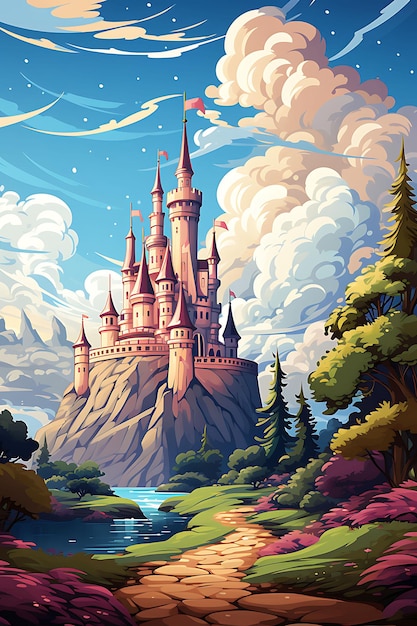The illustration depicts a grand, fantasy-inspired castle, perched majestically on a rocky base that extends down to the edge of a crystal blue body of water. The scene is enclosed in a vertical rectangle. The castle, slightly left of center, stands tall with several cylindrical towers adorned with pointed spires and flags, the tallest featuring a prominent lookout. The stone path, paved with natural circular stones, winds alongside lush green grass on the right of the water, disappearing behind vibrant purple bushes and tall trees. On the left side of the water, another stretch of green grass and short trees extends out of the image.

In the distance, the landscape continues with more green bushes and trees. The background is dominated by an ethereal sky, filled with a blend of white and brown clouds and sprinkled with white dots, possibly stars, suggesting a fantastical, twilight hour. Above the castle, larger mushroom-like clouds loom, adding a surreal element to the scene. Intriguingly, a mysterious gray form with spikes suggests the presence of a dragon, partly visible on the left. The entire composition evokes a whimsical, dream-like atmosphere, reminiscent of a fantasy realm.